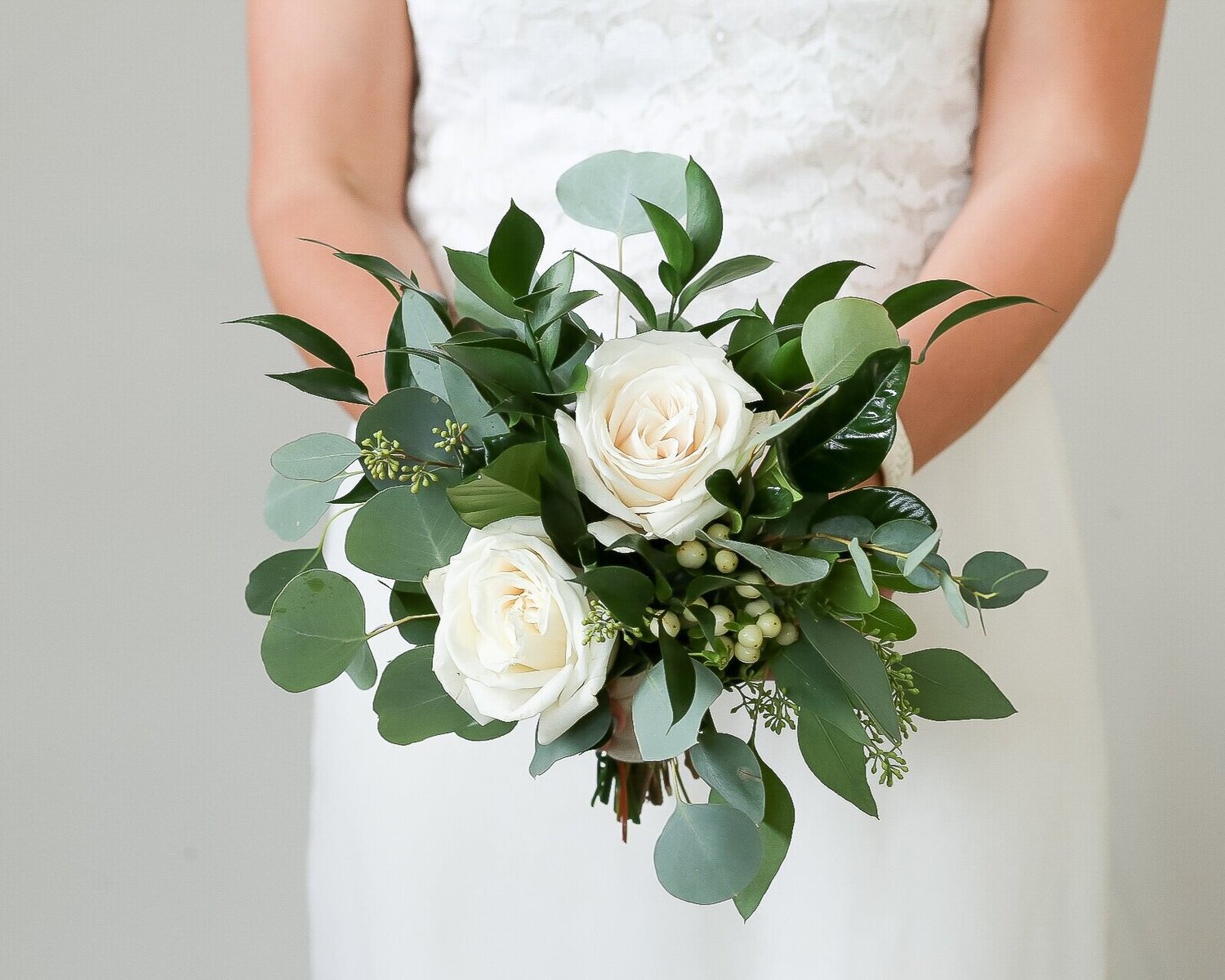This professionally taken, large square photograph features a close-up of a bride’s midsection, showing her from the chest down to the hips. She’s wearing a sleeveless white dress with lacy details above the midsection and a smooth silk-like fabric below. The focus of the image is the bouquet she holds in front of her, composed of two large off-white roses, surrounded by dark green lush leaves and tiny green circular inserts that resemble small pods or berries. Her tannish-pink bare arms frame the bouquet, emphasizing the intricate floral arrangement. The background is a solid light gray, creating a clean and elegant backdrop that draws full attention to the detailed, vibrant bouquet and the luxurious texture of the dress. The overall composition and sharp focus on the bouquet suggest this might be a professional photo for showcasing bridal floral arrangements.